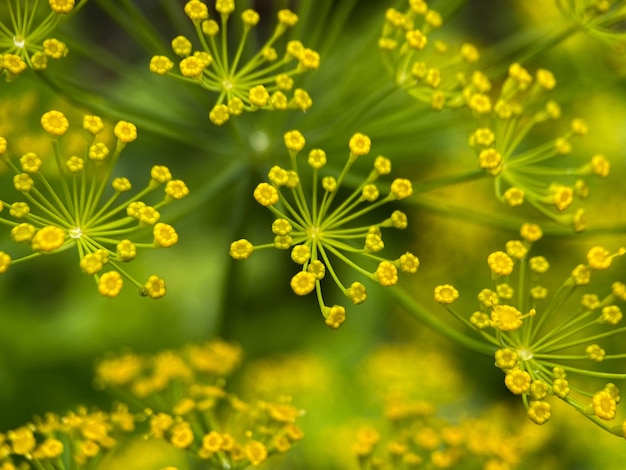This is a detailed macro photograph capturing the intricate structure of a nature scene featuring small, delicate yellow flowers. Each flower, no larger than the head of a needle, is set at the tip of a slender, lime green stem. Approximately 15 to 20 of these tiny flowers branch out from each main stem in a radial fashion, resembling the structure of dandelions but distinctly different. The primary focus is on the cluster of flowers in the center and upper portion of the image, with the background showing similar flowers more softly blurred. The vibrant lime green stems transition gracefully into these minute, radiant yellow flower tips, creating a striking contrast that emphasizes the delicate beauty of this plant. The blurred background enhances the depth of field, leading the viewer's eye to the intricate details of the flowers in the foreground, captivating with their precise and orderly arrangement.